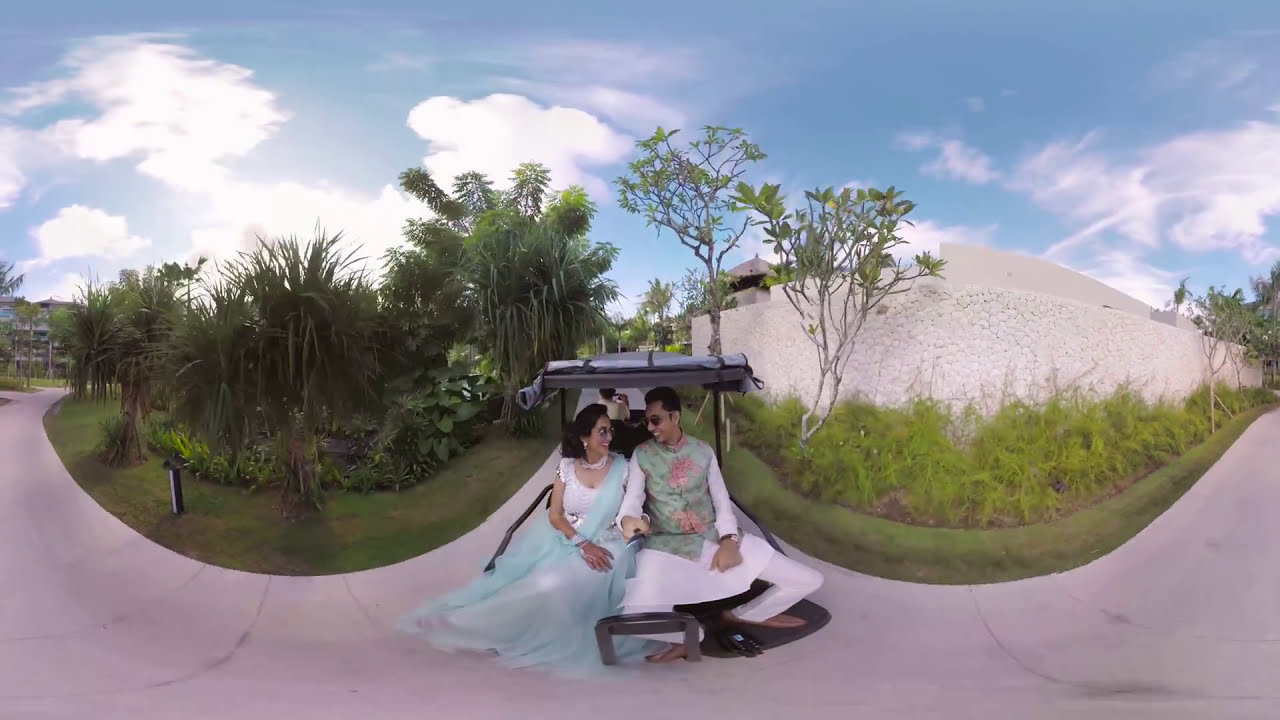In this detailed panoramic photograph taken outdoors, the focus is on a very happy couple seated centrally, facing the viewer. The man, situated on the right, and the woman, on the left, are dressed in traditional attire that may signify a special occasion, possibly their wedding day. The man is wearing white long pants and a greenish vest with pink floral decorations over a longer white shirt. The woman complements him in a beautiful white dress with a light blue or turquoise transparent overlay, accessorized with a white necklace and bracelet. Both have dark hair and are sporting sunglasses, smiling and looking at each other intimately.

They sit close together on a seated structure, which could be a bench or a tram with a gray canopy over their heads. The surroundings are lush and well-manicured, suggestive of a hotel property or resort. On the left side, there is a variety of green trees and bushes, contributing to the semi-tropical ambiance. The paved area in front of them, possibly a sidewalk or road, is white or light-colored, leading through the scenic background. On the right, a white wall suggests a nearby building, possibly a hotel or residence, framed by more greenery. The upper half of the image is dominated by a picturesque sky with wispy clouds dispersed against a blue backdrop, hinting it might be close to sunset. Overall, the photograph captures a serene and joyful moment enveloped in a beautiful, well-manicured outdoor setting.